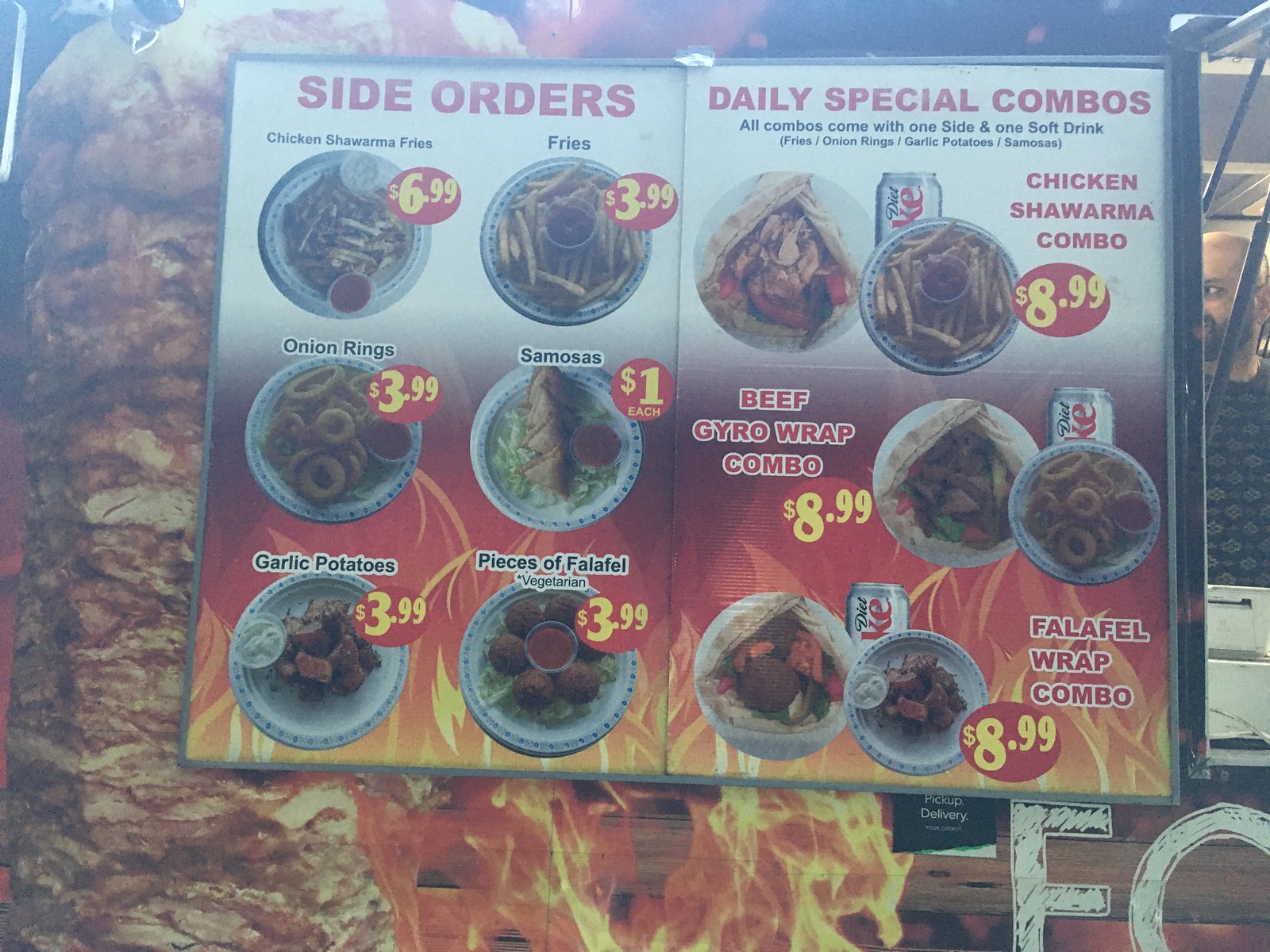The image features a laminated menu printed on paper, displayed open to reveal two pages. The top part of the menu has a clean, white background, transitioning into a reddish-orange hue in the middle, and transforming further into a yellowish color at the bottom. The design includes illustrations of grass leaves rising up from the bottom, adding a natural element to the vibrant backdrop.

On the left page, in bold red letters at the top, the caption "Side Orders" is highlighted. Below, a variety of side dishes are listed:

- Chicken Shawarma Fries - $6.99
- Fries - $3.99
- Onion Rings - $3.99
- Samosas - $1 each
- Garlic Potatoes - $3.99
- Falafel (Vegetarian) - $3.99

The right page showcases the "Daily Special Combos" in equally prominent red letters. The text explains that all combos include one side dish and one soft drink, offering options such as:

- Fries
- Onion Rings
- Garlic Potatoes
- Samosas

The combo meals listed are:

- Chicken Shawarma Combo - $8.99
- Beef Gyro Wrap Combo - $8.99
- Falafel Wrap Combo - $8.99

Accompanying each menu item are images of the dishes, primarily presented on white plates adorned with intricate designs. The images give a visual representation of the meals, enticing potential diners.